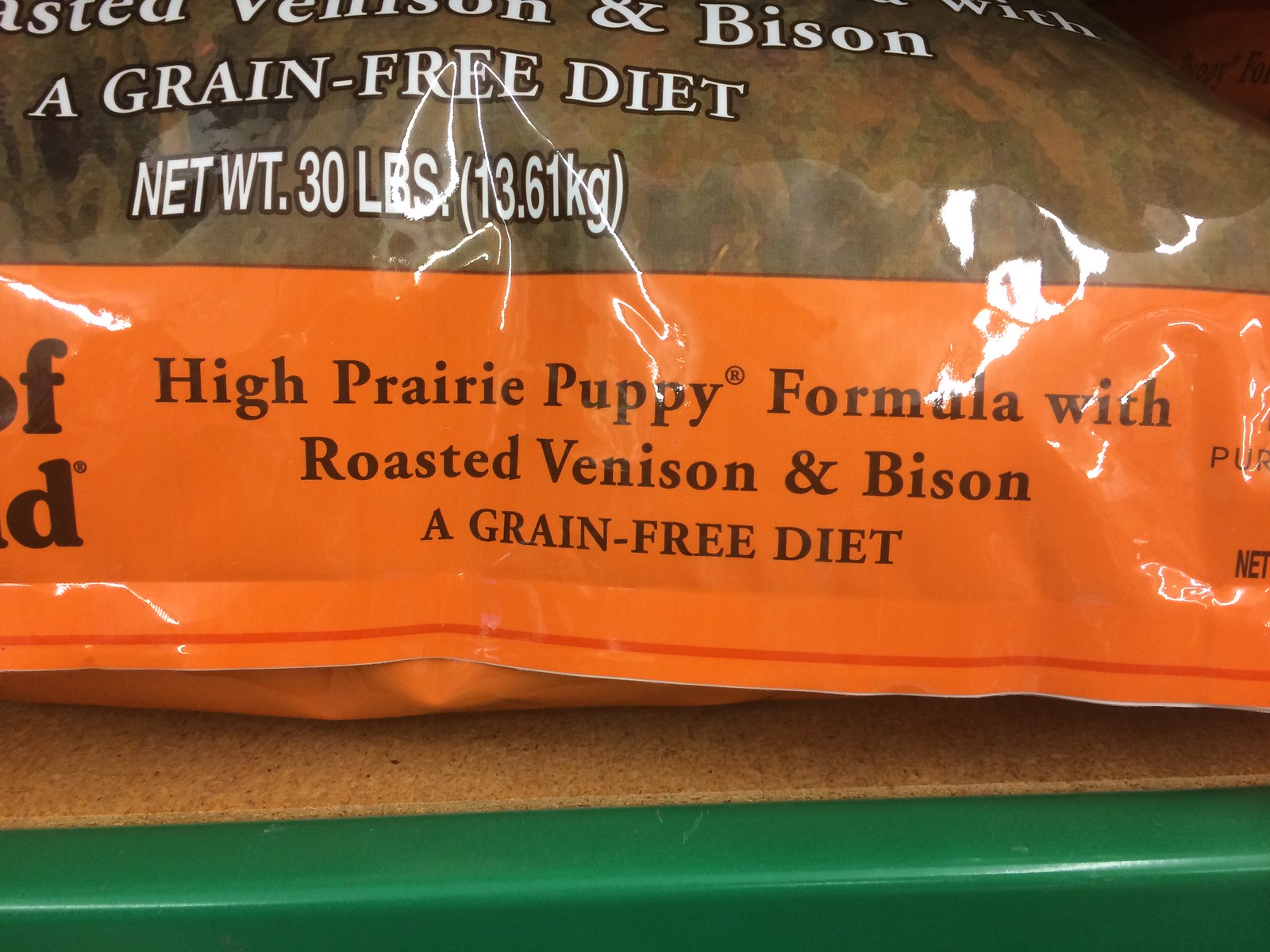The image depicts the lower section of a dog food packaging. Dominating the top part of the image, the text boldly reads "A Grain-Free Diet." Below this, it specifies the net weight as 30 pounds (13.61 kilograms). The product is identified as "High Prairie Puppy Formula with Roasted Venison & Bison," reiterating its grain-free nature. Additionally, there is an illustration of a Dalmatian puppy characterized by its distinctive white coat adorned with black spots. The color scheme of the packaging incorporates tones of oranges and browns, adding warmth and earthiness to the design.